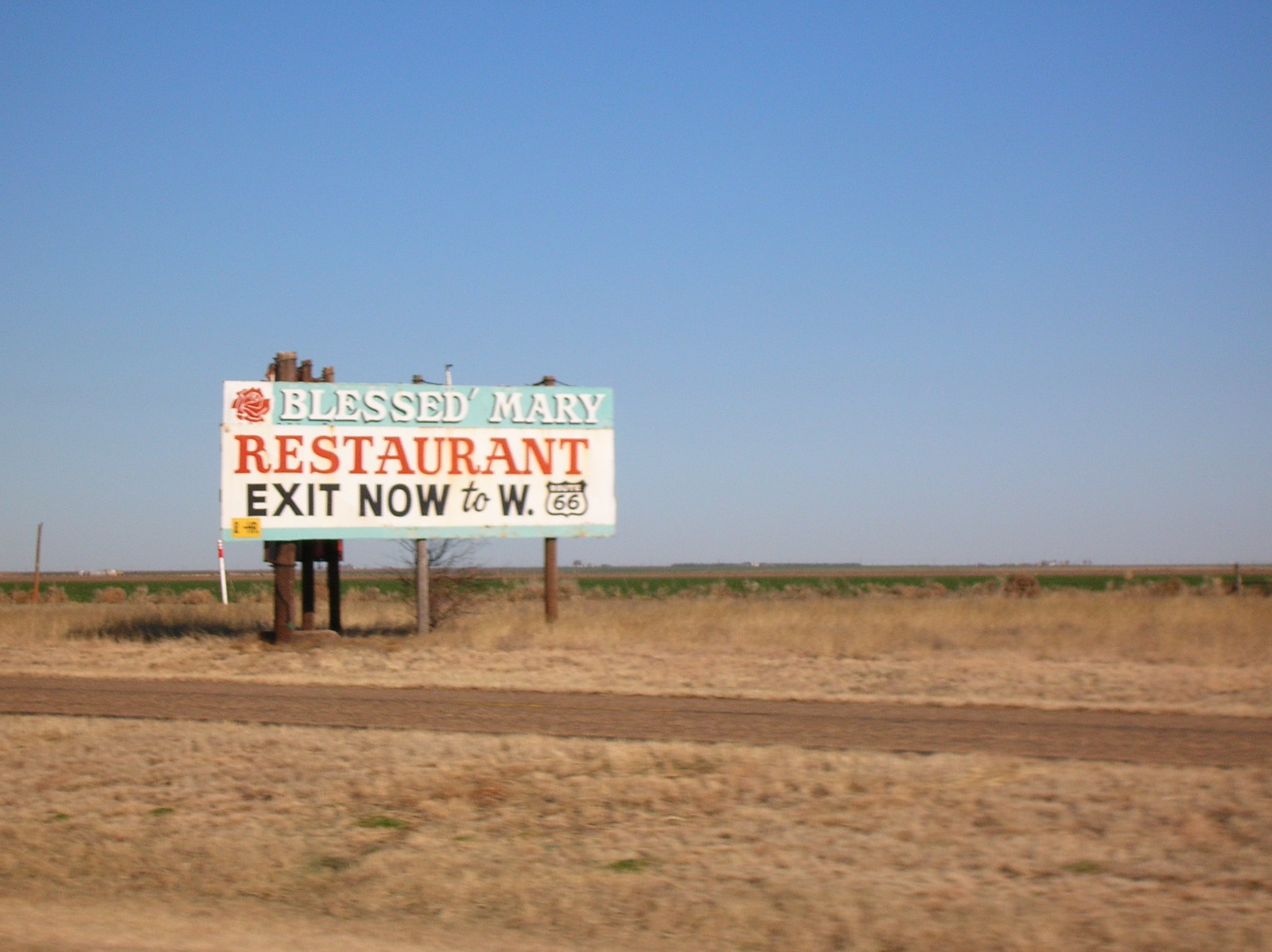The image showcases a scenic rural road dominated by a clear blue sky that gradually lightens near the horizon. In the background, a mix of green and brown fields extends outward, with sparse vegetation, including patches of scrubby grass and perhaps one bush. A prominent white sign, held up by wooden pegs, stands by the roadside. The sign features a striking red rose at the top left and contains text in various colors: a light blue rectangle with white text reading "Blessed Mary," followed by "Red Restaurant" in bold red letters, and "Exit Now to W Route 66" in black letters. The image captures a dirt road flanked by fields, hinting at its proximity to the iconic Route 66. The overall scene suggests an older, slightly filtered photograph with a nostalgic, rustic charm.